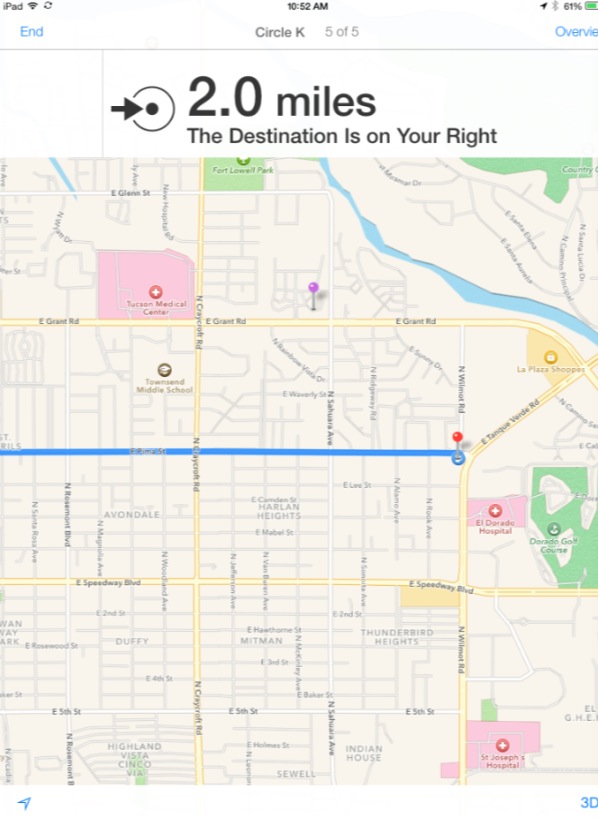The image depicts a person navigating a map on their iPad. The detailed user interface includes the word "iPad" in small black lettering on the top left. To its right, a signal bar is present along with an icon of two arrows pointing towards each other. Further right, the time is shown as 10:52 a.m., accompanied by a black arrow, a grayed-out Bluetooth symbol, and a battery indicator displaying 61% with a small green bar.

In the center, the screen shows "Circle K" with a rating of five out of five stars. On the left of this label, a blue button reads "End," while on the far right, partially obscured, is the word "Overview," with the "W" slightly cut off.

The map section provides the navigation details the user is interested in. A blue pin marks the destination, and a blue line indicates the suggested route. At the top of the map, it says "2.0 miles," and just below that, in black lettering, it instructs that the destination is on the right. The map is fully colored and clearly outlines the path.